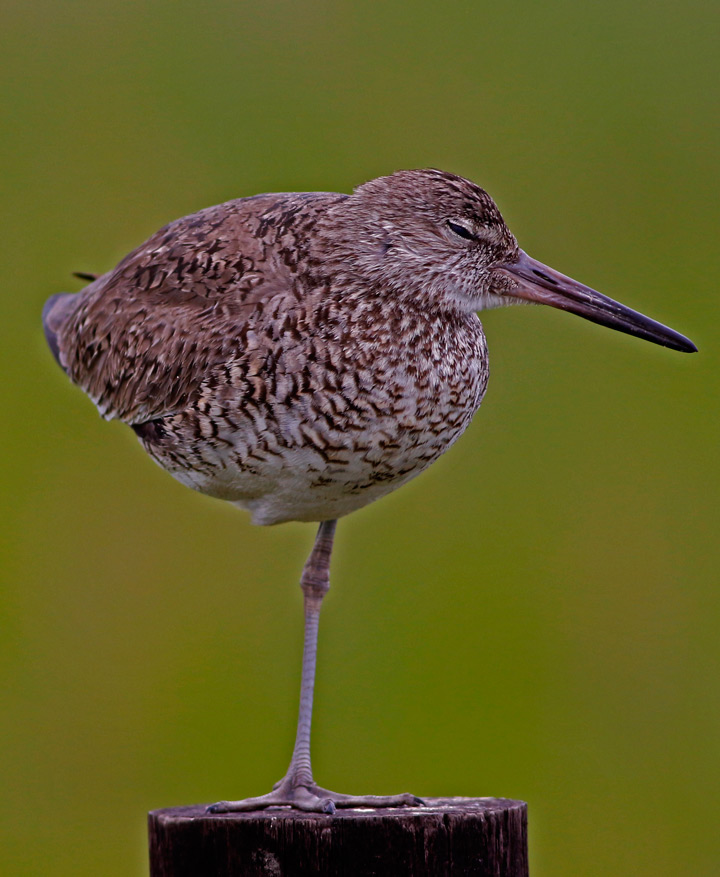This photograph captures an extreme close-up of a bird standing on a rounded wooden stump, likely at a beach or outdoor setting. The background is a blurred green with slight yellow tints, giving the impression of foliage. The bird is in a resting posture, standing on one leg, which appears to be three to four inches long in scale. Its eyes are half-open, half-closed, suggesting it may be relaxing or sleeping. The bird features a very long beak that points downwards, and it is facing to the right. Its plumage is a mix of brown across its top and yellow on its underside, with streaks of brown where its feathers meet, creating a multicolored, rounded belly. The beak, leg, feet, and body share similar splotches of brown, tan, and white. The photo, taken during the daytime, does not contain any text, people, or date markings, emphasizing the solitary beauty of the bird against the serene outdoor backdrop.